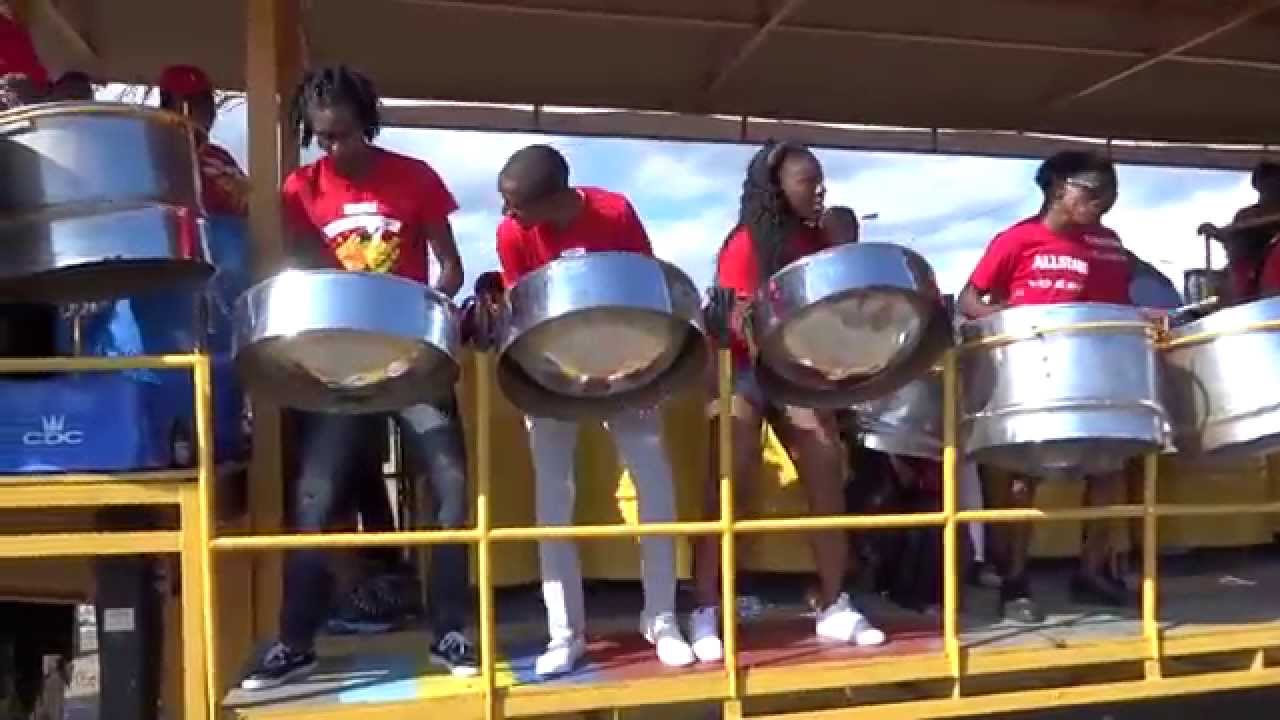In this lively image, we see a close-up of a vibrant steel drum band comprising four black musicians, three men and one woman, all attired in matching red shirts. Positioned on a yellow-railed platform with an overhanging tiled ceiling against a backdrop of blue sky, the group exudes energy as they play their shiny steel pedal drums. To the left, a blue sign with a crown and the "CDC" acronym is visible. One of the men, dressed in blue jeans, is playing a distinctive set of double drums, while the other three musicians, including the bare-legged woman and a man in white pants, each have single steel drums. The drums vary in size, with some resembling half steel barrels and others appearing as several-foot-diameter rings. Their shirts are emblazoned with white lettering, with one shirt distinctly reading "All Stars." Together, they create a harmonious blend of rhythm and melody, filling the air with their powerful, resonant tunes.